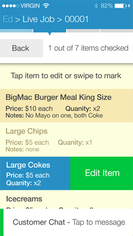The image depicts the screen of a mobile phone displaying a food order summary. The top section of the screen has a blue background and includes several status indicators: 

- In the top left corner, the text "Virgin" is displayed, indicating the mobile carrier Virgin Mobile.
- A Wi-Fi icon is positioned slightly to the right.
- On the top right, the battery percentage reads "82%", accompanied by a battery icon.

Below this blue section, the screen transitions into a white rectangular area containing order progress information: "1 out of 7 items checked."

The primary content below this includes a list of checked food items in a pale tan colored box with black text, which provides interactive options through editing or marking. The list consists of:

1. **Big Mac Burger Meal (King Size)**
   - Price: $10 each
   - Quantity: 2
   - Notes: No mayo on one, both with Coke

2. **Large Chips**
   - Price: $5 each
   - Quantity: 1

3. **Large Cokes**
   - Price: $5 each
   - Quantity: 2
   - Option to edit item

4. **Ice Creams**
   
The layout and interactive elements suggest that this is a food order application, possibly a service like DoorDash or Uber Eats.